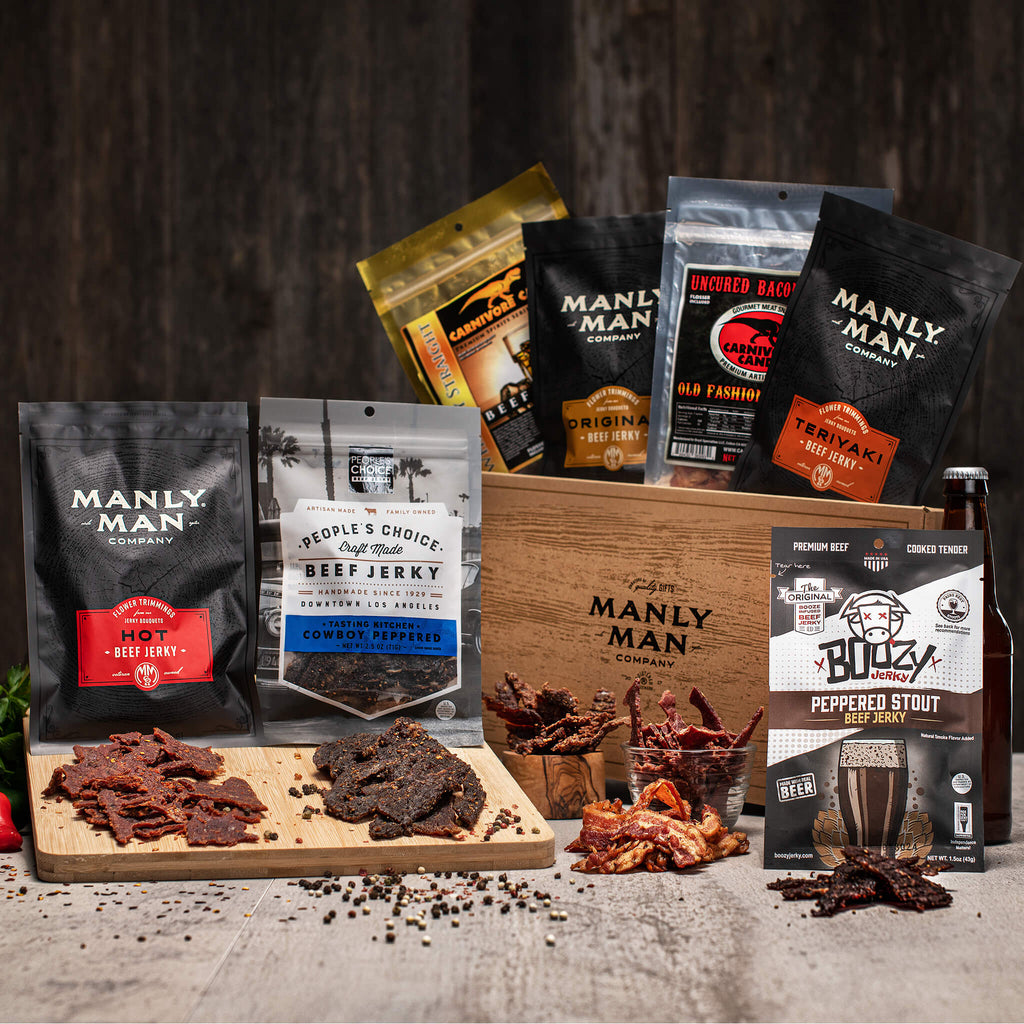The image is a detailed advertisement for Manly Man Company jerky products, featuring a variety of beef jerky packages. The backdrop of the image is a dark wooden wall, with a wooden table beneath it. Centrally located is a cutting board showcasing two types of jerky: on the left, piles of hot beef jerky in a black foil package marked by a reddish-brown hue with flames and a man printed on it; on the right, People's Choice Craftmade Beef Jerky, Cowboy Peppered, in a gray foil package with jerky pieces in front of it. 

Adjacent to the cutting board is a branded wooden crate with "Manly Man Company" burned into it, containing four jerky varieties in visible pouches. These are (from left to right): Carnivore Camp's Uncured Bacon Jerky in a silver pouch, Manly Man Company's Original Beef Jerky in a black bag, Carnivore Camp's Old-fashioned Uncured Bacon Jerky in a silver pouch, and Manly Man Company's Teriyaki Beef Jerky in a black bag. In front of the crate are additional piles of jerky, including some uncured bacon jerky.

To further the assortment, the right side of the display features a glass with ripple patterns filled with jerky, and a bag of Boozy Jerky, Peppered Stout Beef Jerky, characterized by a cow’s head with X’s for eyes and the tagline "Made with Beer." This package is accompanied by a picture of a dark beer bottle. The entire setup is accented by scattered peppercorns and spices, lending an artisanal feel to the advertisement. The overall composition, set against a rich, dark wooden background, emphasizes the robust, hearty nature of Manly Man jerky products.